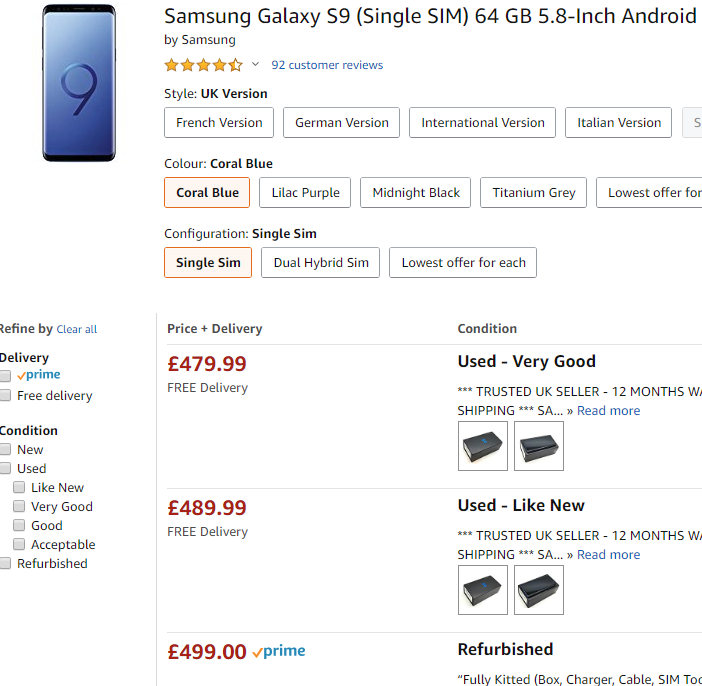A detailed caption for the given image could be:

"A screenshot from a website displayed on a Samsung mobile phone is shown in the upper left-hand corner. The phone, which appears sleek in gray and black, features a prominent '9' on its back. To the right of the image, the text 'Samsung Galaxy S9' is clearly visible, with additional details in parentheses indicating it as a 'Single SIM,' model with '64 GB' storage and a '5.8-inch Android' display. Below, the text 'by Samsung' appears in a smaller font, followed by a star rating just above four stars, with the fifth star partially shaded. Further down, '92 customer reviews' is highlighted in blue. The 'Style' is noted as 'UK version,' and the 'Color' is specified as 'Coral Blue,' with alternate color options including 'Lilac Purple,' 'Midnight Black,' and 'Titanium Gray.' 

Continuing lower, a partially visible element labeled 'alpha 4' is mentioned. Available versions include 'French version,' 'German version,' 'International version,' and 'Italian version,' with one more version hidden out of view. The configuration options are listed as 'Single SIM' and 'Single SIM, Dual Hybrid SIM,' with lowest offers for each. Pricing information indicates the lowest offer in black text as 'price plus delivery,' with the price noted as '€479.99' in red, which includes 'free delivery' in black text. The condition of the phone is described as 'used very good.' Another price listed is '€489.99' for a 'like new' condition, also with free delivery. Lastly, the highest offer is '€499' for a 'refurbished' unit, marked with a Prime check for availability."